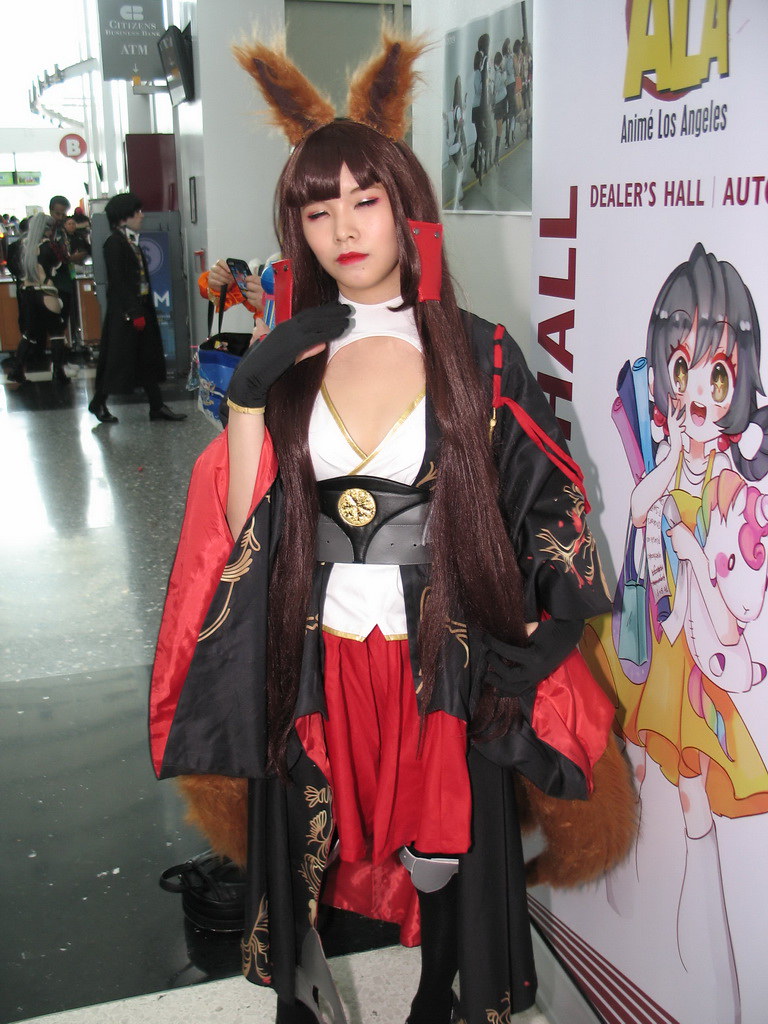In this well-composed photo taken at the Anime Los Angeles (ALA) Dealers Hall, a young woman of Asian descent stands out in a detailed and elaborate cosplay ensemble. She showcases a pair of tall, fuzzy, brown ears atop her head, set against her long, dark hair with bangs. Her hairstyle is complemented by red square structures resembling clips on each side of her head, possibly to secure or accentuate her hair. Her makeup is striking, with silver eyeshadow rimmed by red-pink hues that extend beneath her bottom lashes, paired with bold red lipstick.

She dresses in a white blouse featuring a distinctive cutout shaped like a fan that arches from the top of her chest and angles down to her breastbone. Gold piping adds a rich accent along the blouse's edges. Below this, a large black belt with a central gold round emblem cinches her waist, aligning with the cropped blouse adorned similarly with gold piping. A deep red long skirt flows from her waist, coordinated with her black gloves and a black cape that flaunts Chinese designs on the sleeves and a red lining. Notably, the base of her outfit mimics the furry texture of her headpiece. 

Standing in a doorway beside a sign bearing an anime character with the text "ALA, Anime Los Angeles Dealers Hall," she is captured with her right hand delicately touching her neck. Other cosplayers and a hint of light streaming through a window can be seen in the background, adding depth to the setting. This photograph not only captures her detailed costume but also reflects the vibrant atmosphere of the convention.